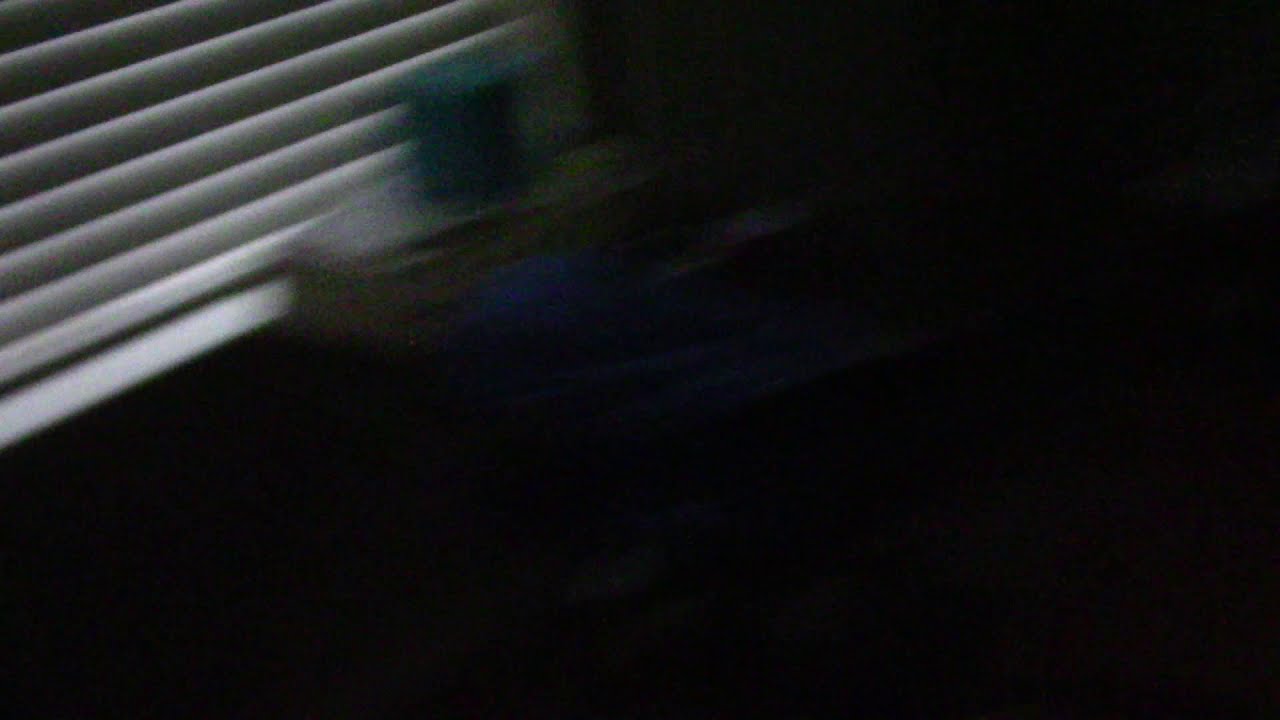This image is a close-up of white window blinds, fully pulled down and closed, with a faint light filtering through the slats. Framed in the upper left corner, the blinds and the window indicate it's nighttime outside, contributing to the overall darkness of the room. Adjacent to the window is a dresser, partially visible and blending into the dark background. A blurry, indiscernible object, likely blue and white, stretches across from one end of the blinds to the middle. Although the room is very dark and most details are fuzzy, the presence of the blinds and the mysterious blue object are the most discernible elements in this image.